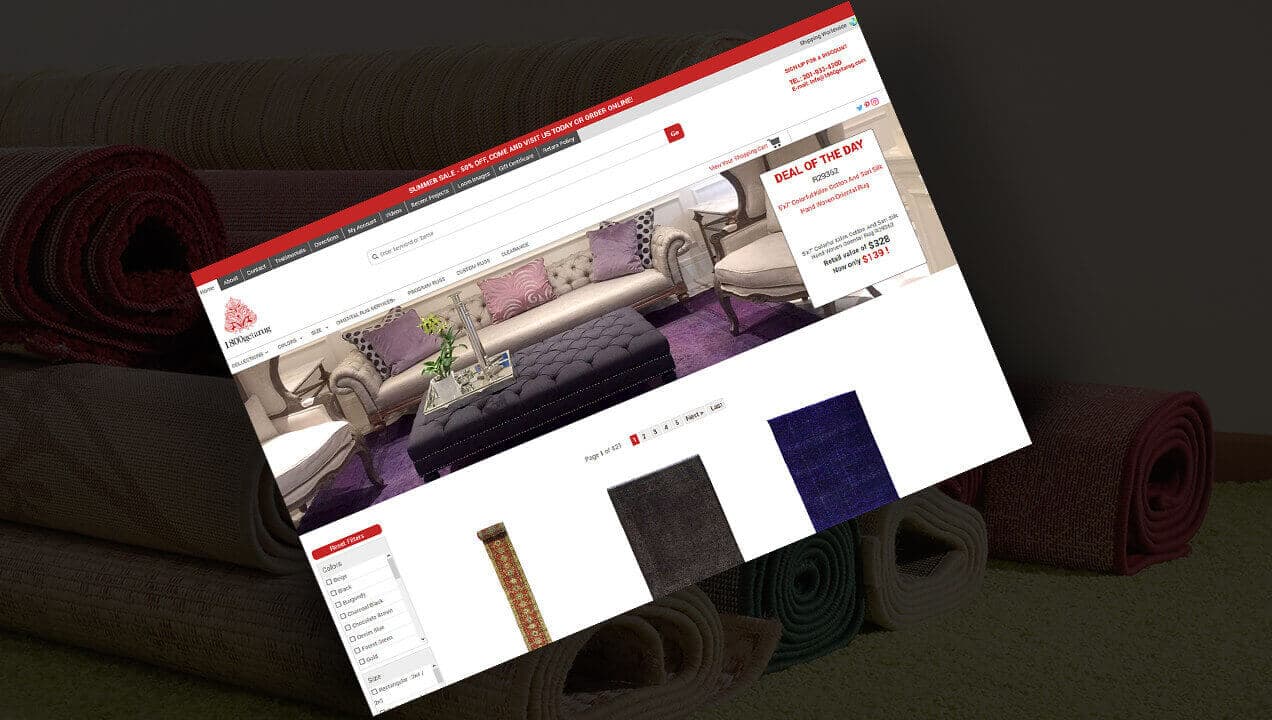The image features a heavily grayed-over photograph of what appears to be rolled Persian rugs stacked on top of each other, forming a muted, textured background. Superimposed over this backdrop is a tilted, diagonal view of a website's homepage. The upper right corner of the website aligns with a point roughly two-thirds from the right edge of the image, while the bottom left corner extends to about one-third from the right edge along the bottom. The website is presented with a dramatic diagonal tilt.

The top bar of the website is prominently red, displaying a banner that presumably advertises a "Summer Sale" with discounts of "50%" or a similar figure, accompanied by a call to action like "Visit Us Today." The navigation bar below this prominently features tabs, though their labels are not fully discernible, likely including "Home," "About," "Contact," "My Account," and possibly "Gift Certificate." However, the text and overall resolution of the website appear reduced and somewhat pixelated, making finer details challenging to distinguish.